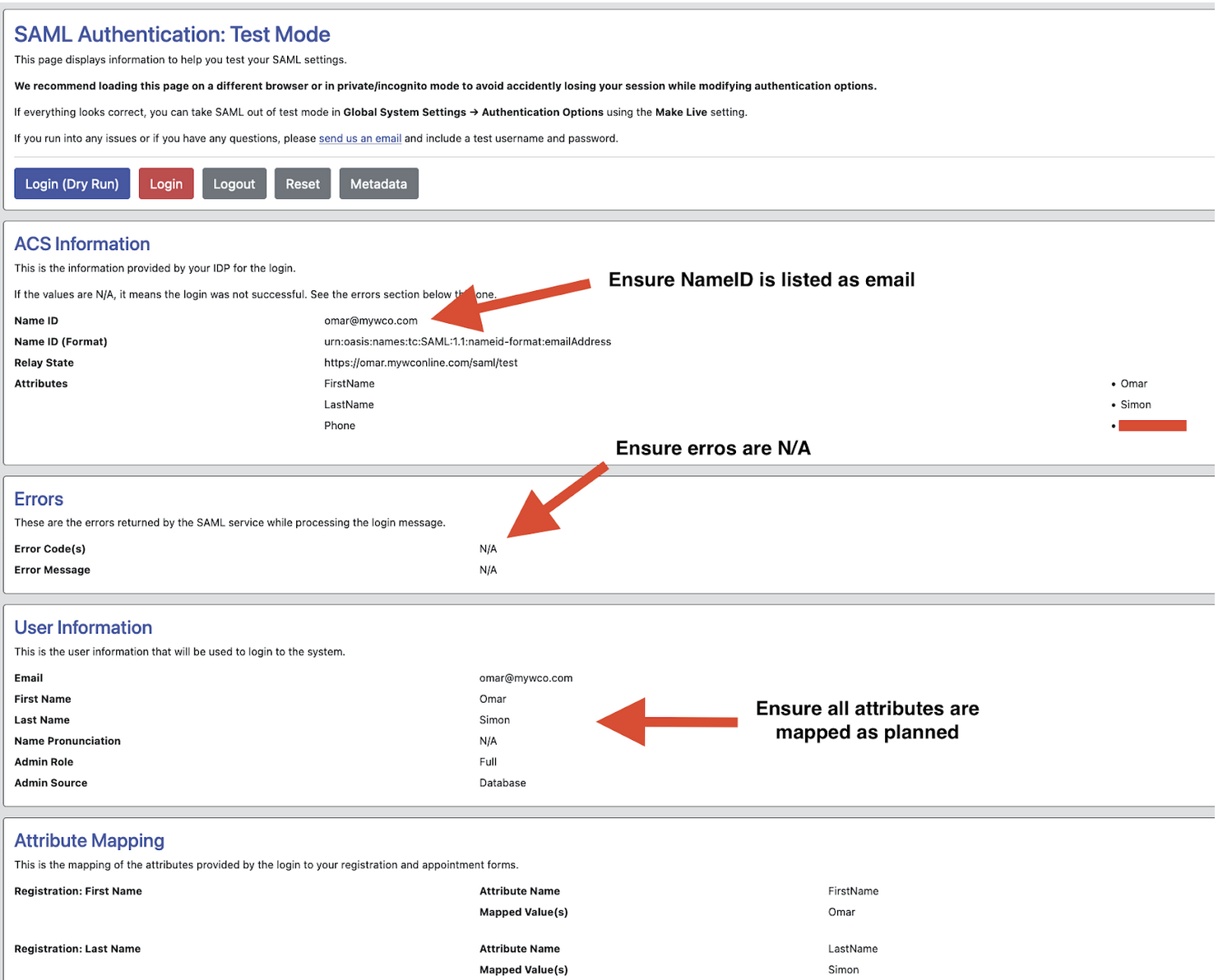**Detailed Caption:**

The image showcases a webpage titled "SAML Authentication Test Mode." The primary purpose of this page is to assist users in testing their SAML (Security Assertion Markup Language) settings. Users are advised to open this page in a different browser or use an incognito/private mode to prevent session loss during authentication option modifications. Should everything appear correct, SAML can be taken out of test mode by adjusting the global system settings under the authentication options using the "Make Live" settings. For any issues or questions, contact support via email, including a test username and password for troubleshooting.

The page features several buttons: "Login" and "Dry Run" in red, "Log Out" in gray, and "Reset" and "Metadata" in unspecified colors. Below the instructional text, there's a section labeled "ACS Information," followed by another section, "Name ID," with a red arrow pointing to an email address, suggesting that the "Name ID" should be listed as an email. Another distinct section is labeled "Errors," with a red arrow pointing to "N/A," indicating that no errors should be present (denoted as "N/A"). Additionally, in the "User Information" section, there is an arrow pointing to the last name "Simon," indicating that all user attributes should be mapped as planned.

The text on the page is primarily in black, with red arrows highlighting critical information. Various buttons stand out with their distinct colors, aiding in the navigation of the page and functionalities related to SAML authentication testing.